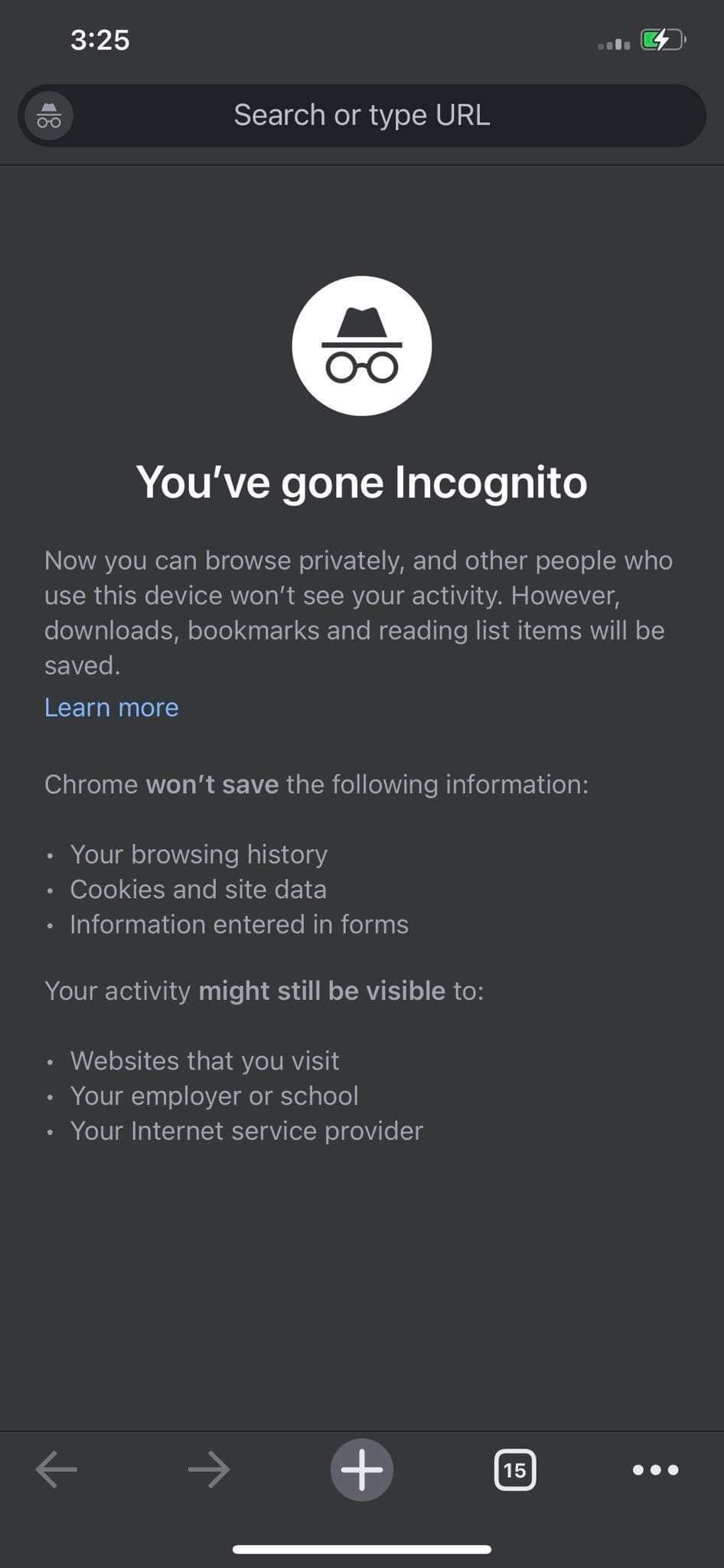A smartphone screen displays a new incognito browsing session in the Google Chrome browser. The screen shows the time as 3:25, with indicators for cellular signal strength and a half-full, charging battery at the top. Within the browser, the search bar reads "Search or type URL," while just beneath it, a circular icon featuring a hat and glasses announces "You've Gone Incognito." The screen explains that you can now browse privately, and other users on this device won't see your activity. However, downloads, bookmarks, and items in the reading list will still be saved. The message highlights that Chrome won't save your browsing history, cookies, site data, or information entered into forms. Still, your actions may be visible to websites you visit, your employer or school, and your internet service provider.

At the bottom of the screen, navigation icons are visible, including left and right arrows, a plus sign within a circle, the number "15" in a square, and a vertical three-dot menu indicator. Below these icons, there is a white navigation bar in the center. The color scheme of the screen consists primarily of shades of white, black, slate gray, and green, with some blue accent text for the "Learn more" link.